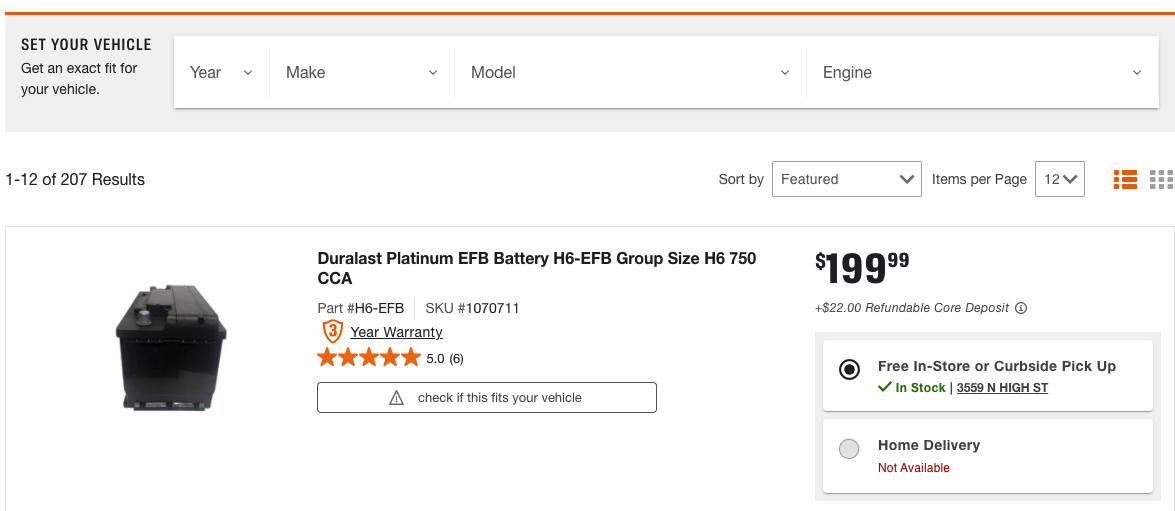This image depicts an auto store's online shopping interface. The screen background is white, with black text set in a left-to-right orientation. The interface prompts users to "Set your vehicle, get an exact fit for" and features a search box allowing selections for the year, make, model, and engine of a vehicle. The current search results indicate 1 of 12 items displayed out of a total of 270 results. 

Users have the option to sort the items and adjust the number of items displayed per page (currently set at 12). There are links for three additional lines and nine dots indicating further navigable options. 

The highlighted product is an image of a battery with the following details: 
- Name: Durablast Platinum EFB Battery HC-EFB
- Group Size: H6 
- CCA: 750
- Part Number: H6-EFB 
- SKU Number: 1070711 

The battery comes with a 3-year warranty and has a 5-star rating based on 6 reviews. Beneath the product description is a button to check compatibility with the user's vehicle. The price is listed at $199.99 with an additional $22 refundable core deposit. 

The product is available for free in-store or curbside pickup—with the stock status confirming availability—at 3559 North High Street. Home delivery is also displayed as an option, although currently not available. The selected option for acquisition is free in-store or curbside pickup.